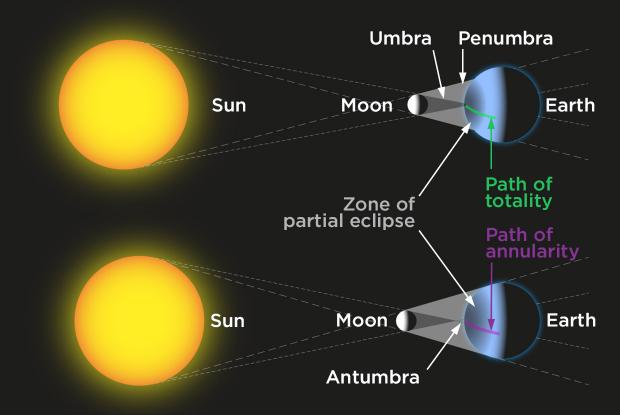This image features a detailed diagram on a black background illustrating the different phases of eclipses. At the top, it shows the sun, moon, and earth aligned to depict a solar eclipse, with annotations for the umbra, penumbra, path of totality, and the zone of partial eclipse. The sun is a bright yellowish orb with an orange perimeter, and arrows indicate the alignment necessary for various eclipse phases. The bottom section highlights the antumbra and features the moon and earth again, showcasing different eclipse stages. The diagram, partly in Spanish, includes terms like "umbra" and "penumbra" and illustrates the path of totality and annularity. This comprehensive chart explains how the sun can be completely or partially obscured by the moon, depending on the observer's location on Earth.